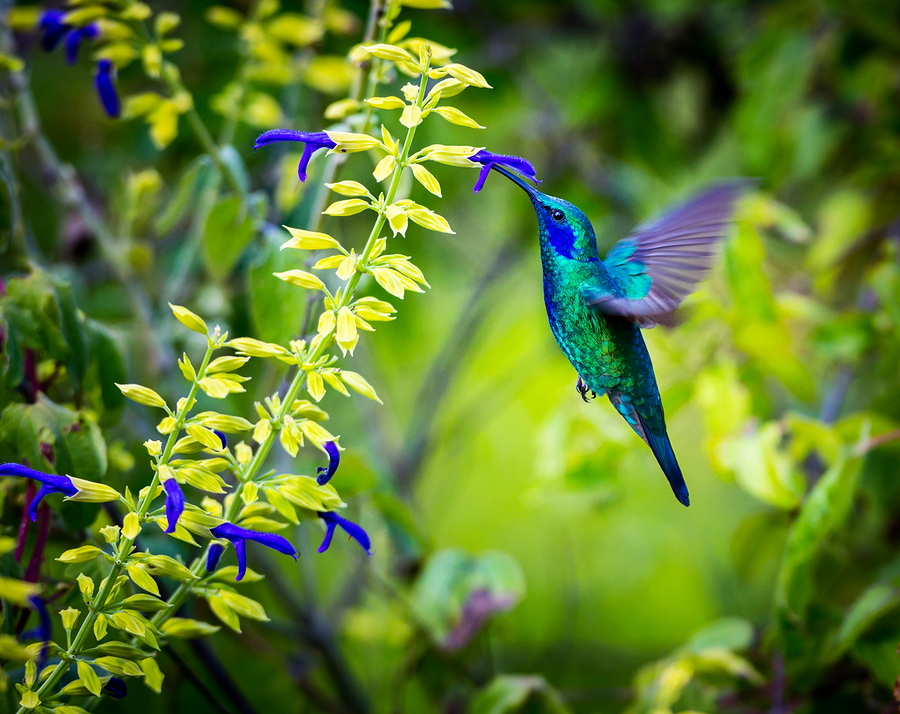The image features a vibrant and sharply focused hummingbird captured mid-flight, hovering as its long blue beak probes a delicate flower. The hummingbird, centered in the frame and flying from right to left, is an exquisite blend of translucent luminescent green and striking blue. It boasts blue under the eyes and belly, with its head and back also shimmering in blue hues. The bird’s wings, a blur in their motion, reveal shades of blue, purple, and green. The tail is distinctly blue with two black stripes.

In remarkable detail, the claws of the hummingbird’s feet and its sharp scales and feathers are visible. The bird feeds from a beautiful, long-stemmed plant adorned with blue petals and green leaves that stretch from the top to the bottom of the image. The background is softly blurred using a bokeh effect, creating a mosaic of yellow, lime green, and hints of blue and purple, suggesting a lush forest or garden scene, likely in spring or summer. The overall image highlights the contrast between the crystal-clear depiction of the hummingbird and the softly out-of-focus greenery behind it, enhancing the vivid beauty of this moment in nature.